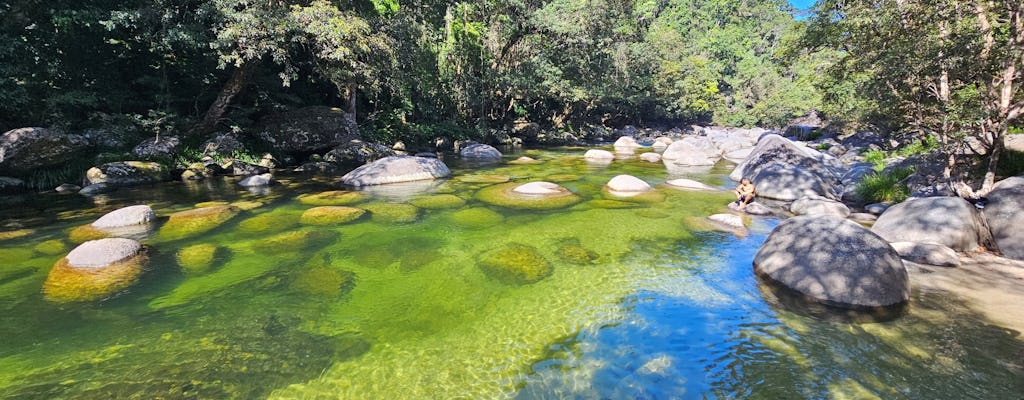This photograph captures an idyllic, sunlit scene of a shallow pond or stream set in a heavily wooded, forested area. The serene body of water is dotted with large, smooth rocks, some half-submerged and others jutting above the surface. The water exhibits a striking gradient, transitioning from a clear, pale blue on the left to a green hue mired with algae throughout the rest. At the bottom, the water reveals a layer of algae. The pond forms a rough circular shape, surrounded by a diverse and lush greenery varying from dark, dense foliage on the left to a sunlit center and right, which is slightly darker. In the distance sits a couple on a rock, the woman leaning back against the man, both enjoying the tranquility and beauty of the day. Behind them, a larger rock hosts a small waterfall cascading gently into the pond. This wide-angle shot encapsulates the peacefulness of this hidden gem, making it a perfect, Eden-like retreat absent of any other human presence.